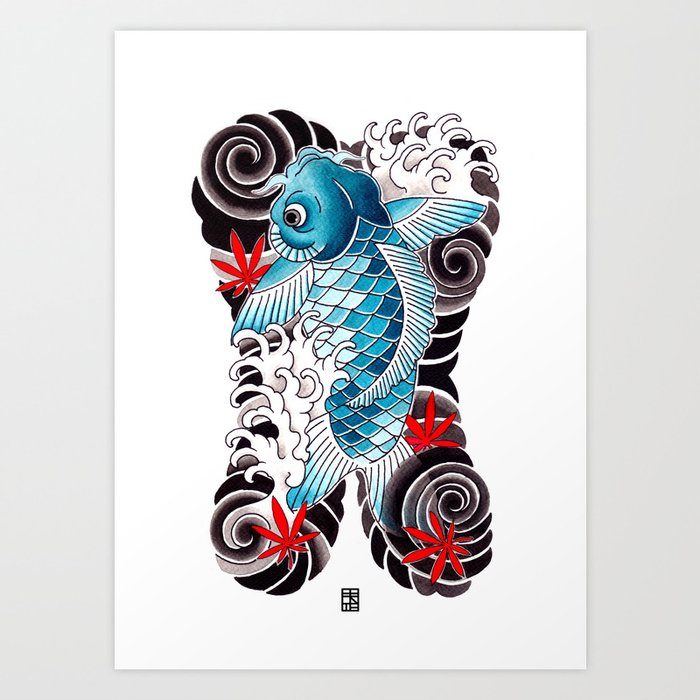This is a detailed illustration inspired by traditional Japanese art, depicting a turquoise blue koi fish, shaded with varying hues of light to darker blues, gracefully navigating through black ocean waves adorned with white foam. The fish, seen from above, has meticulously detailed scales and lighter blue fins, with a prominent fin that stretches along its back, pointing to the right. Surrounding the koi are black swirls with interspersed gray accents, and positioned within this dynamic aquatic scene are four vibrant red Japanese maple leaves, each leaf strategically placed: one at the top left, one at the bottom left, and two near the bottom right. The composition, which could easily be envisioned as a back tattoo, features Japanese lettering at the bottom of the image, all set on a clean white background, underscoring the image's aesthetic with a harmonious balance of color and traditional motifs.